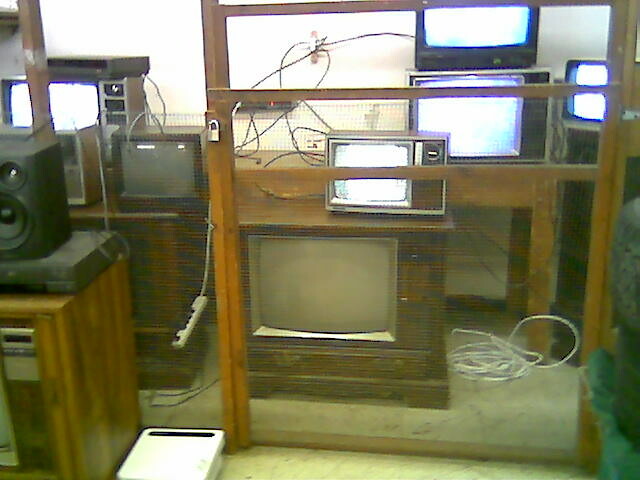In this color photograph taken indoors, we are presented with a scene that appears to be a television repair shop or a used furniture store filled with old televisions. Dominating the foreground is a large, brown wooden console TV with a smaller TV perched on top. To the left, a cropped wooden shelving unit supports a home theater speaker and possibly a CD player or turntable.

Behind this, a chicken wire-style fence with a wooden gate and a silver padlock encases a collection of TVs, some of which are turned on, displaying white static screens. The TVs range in era, from the 1950s to the 1970s, characterized by their bulky, wooden cases, manual dials for changing channels, and cathode ray tubes. The room’s floor is a yellow or beige color, cluttered with extension cords running across the walls and floor.

On the far right, there's a hint of a plant and additional small TVs sitting on shelves. The overall scene is somewhat dimly lit, and the photo's focus is slightly blurred, lending it a retro and nostalgic atmosphere. The wall behind the TVs is white, accentuated by the tangled maze of power cords and a gray VCR, further emphasizing the old-school vibe of the setting.